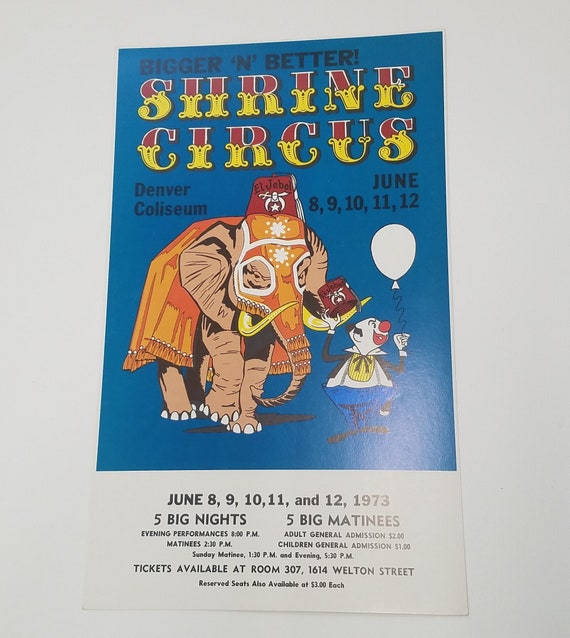The image is a photo of a poster announcing the Bigger and Better Shrine Circus at the Denver Coliseum, taking place from June 8th to June 12th, 1973. The top of the poster features the text "Bigger and Better" in black capital letters, followed by "Shrine Circus" in a vibrant red and yellow font outlined in white, reminiscent of a traditional circus style. Dominating the central area of the poster is an illustration of an elephant adorned in an orange covering, accompanied by a clown. The clown, positioned to the right of the elephant, is depicted holding a white balloon in one hand and a Shriner's hat in the other, with his own hat tipped off. The backdrop of the poster is mostly dark blue, contrasting with the bottom portion that has a white background. Below the main illustration, the poster reiterates the event dates, June 8th to 12th, 1973, and highlights that there will be five big nights and five big matinee performances. Specific showtimes are mentioned but difficult to read. The white section also provides ticket information: tickets can be bought at room 307, 1614 Welton Street, with reserved seats available. General admission is listed as $2 for adults and $1 for children.